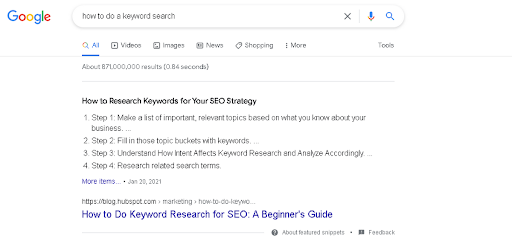Screenshot of a Google Search Query: "How to do a keyword search"

In this screenshot, the Google logo is prominently displayed in the top left corner. Each letter in "Google" is colored distinctively: the first 'G' is blue, the 'O' is red, the second 'O' is yellow, the second 'G' is blue, the 'L' is green, and the 'E' is red. Below the logo, the search bar shows the query "how to do a keyword search."

Underneath the search bar, a navigation menu includes the options: 'All' (selected), 'Videos,' 'Images,' 'News,' 'Shopping,' 'More,' and 'Tools.' The results indicate about 871 million matches, retrieved in 0.84 seconds.

The first search result is an article titled "How to research keywords for your SEO strategy" and lists the following steps:
1. Make a list of important relevant topics based on what you know about your business.
2. Fill in those topic buckets with keywords.
3. Understand how intent affects keyword research and analyze accordingly.
4. Research related search terms.

This article appears on a webpage from HubSpot, specifically at https://blog.hubspot.com/marketing, dated January 29, 2021, with the title "How to do Keyword Research for SEO: A Beginner's Guide."

In the bottom right corner of the screenshot, there is an option to learn more about 'Featured Snippets' and a 'Feedback' link.